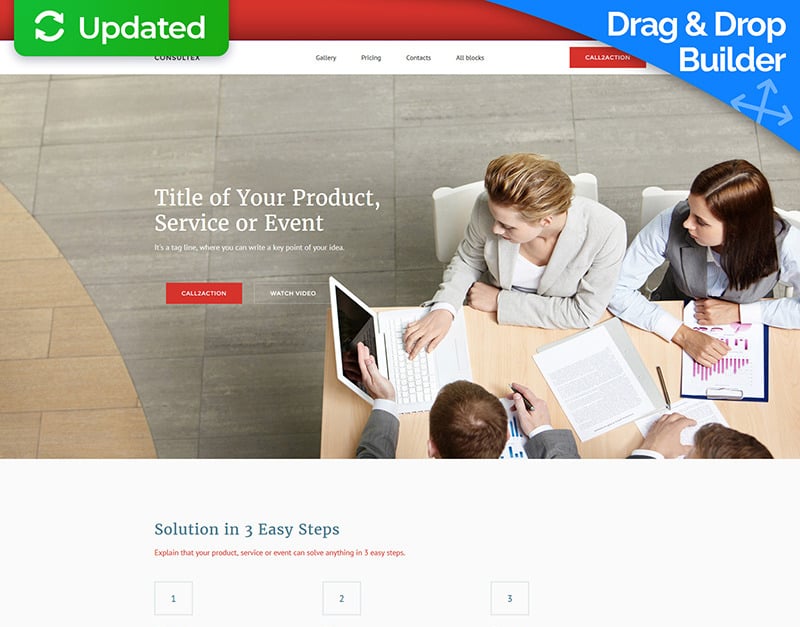The image features a red border at the top. On the left side, a green box partially covers the red border. This green box contains two circular arrows and the word "Updated" on its right side. On the right side of the image, there is a blue section titled "Drag and Drop Builder." Below this title, a menu includes options such as "Gallery" and "Pricing," though two of the items are too blurry to identify. Further down, there's text that reads "Title of Your Product, Service or Event," followed by an unreadable sentence. Below this text, a red button, starting with a "C," is present, and to its right is a gray button labeled "Watch Video." The central part of the image shows a wooden table with two men and two women seated around it. They are focused on a laptop, with papers, folders, and ink pens scattered on the table.